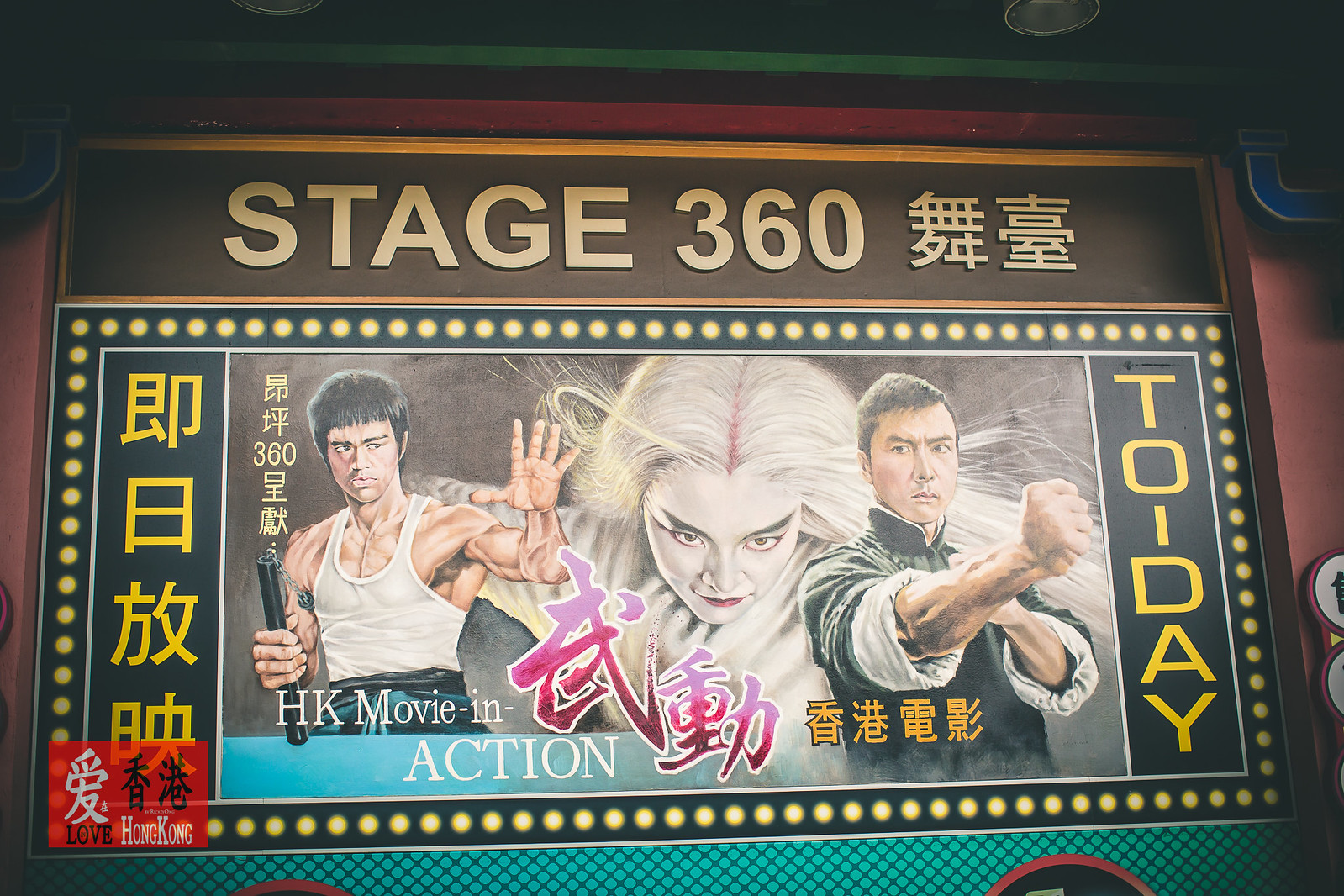The image is a detailed poster for a film displayed at a cinema theater, prominently featuring a brown sign at the top that reads "Stage 360" in gold letters alongside some Chinese characters, suggesting it could be the theater's name. Below this sign is a vibrant, horizontal drawing with distinct cartoon, painted figures. On the left side of the poster, Bruce Lee is depicted in a white tank top, holding a nunchaku in one hand while raising the other, looking to his left with a serious expression. At the center of the image stands a woman, possibly a sorceress, with an entirely white appearance, from her makeup to her hair, and her arms are open wide. To the right, Donnie Yen, dressed in traditional Chinese clothing, appears with clenched fists, also in a serious pose, looking to his right. The left side of the image contains yellow Chinese characters, while the right side displays English text stating "today." The entire poster is framed by graphic representations of light bulbs, adding a dramatic and vintage theater aesthetic to the overall design.